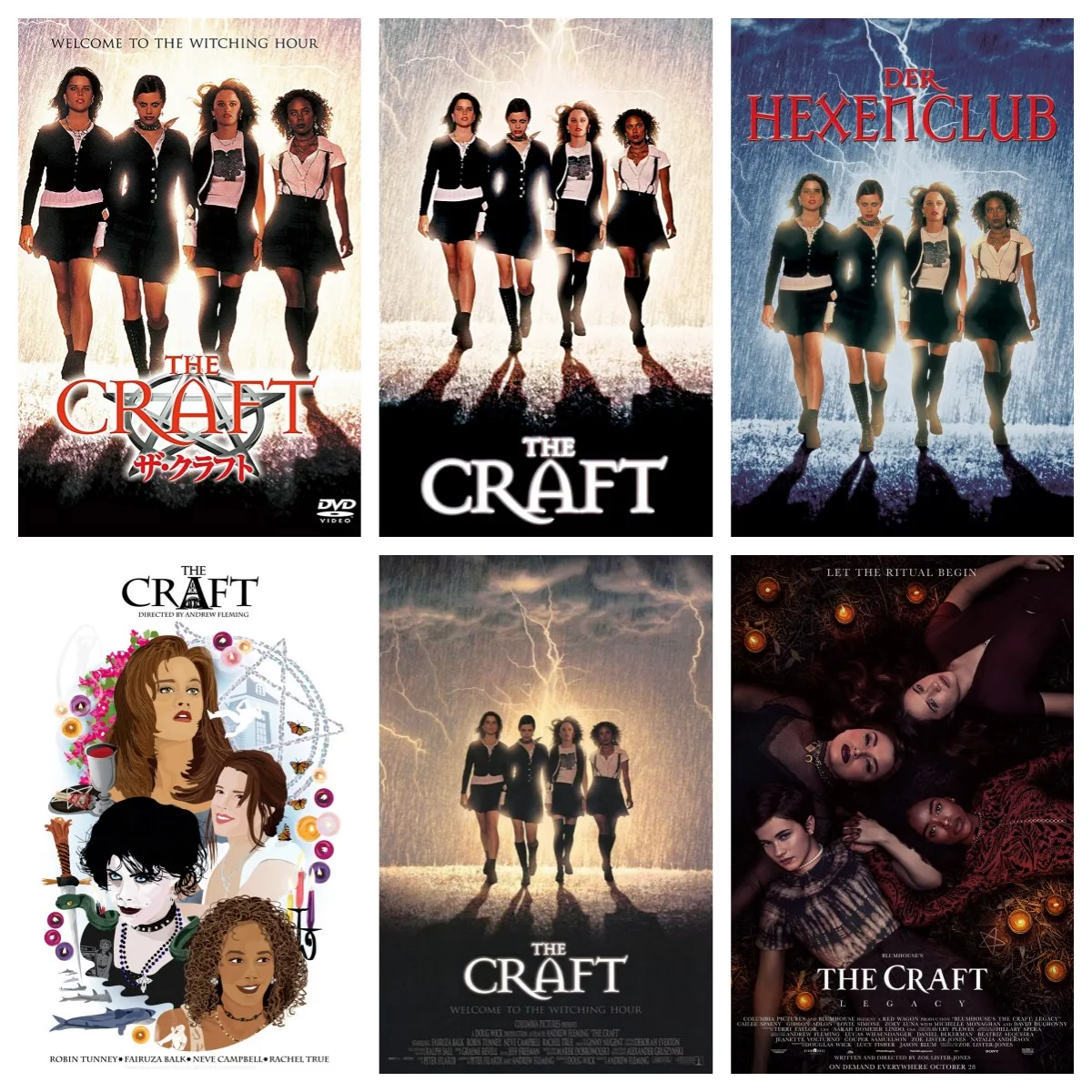The image features six distinct movie posters for "The Craft," arranged in two rows of three. Each poster prominently displays four teenage girls in school uniforms, exuding a serious demeanor. In most posters, the girls are depicted walking side-by-side with a dramatic background, often highlighted by a lightning-filled sky. The top left poster includes the tagline, "Welcome to the witching hour," and shows the girls in black skirts and thigh-high socks against a backdrop of yellowish lightning streaks. The central image on the top row maintains this design but without the tagline, while the top right poster, titled "Der Hexen Club," presents the same scene with a bluer, cloud-filled sky.

The bottom row starts with an animated version of the group on the bottom left, featuring a more cartoonish style where the characters are surrounded by mystical elements like snakes and cauldrons. The middle poster on the bottom mirrors the lightning-struck design from the top row, keeping the dark, intense vibe. The final poster on the bottom right, titled "The Craft: Legacy," shifts dramatically, showing the girls lying down in a cluster with their heads together, surrounded by candles forming a hexagon. The tagline, "Let the legacy begin," appears at the top, suggesting a continuation or sequel to the original film.